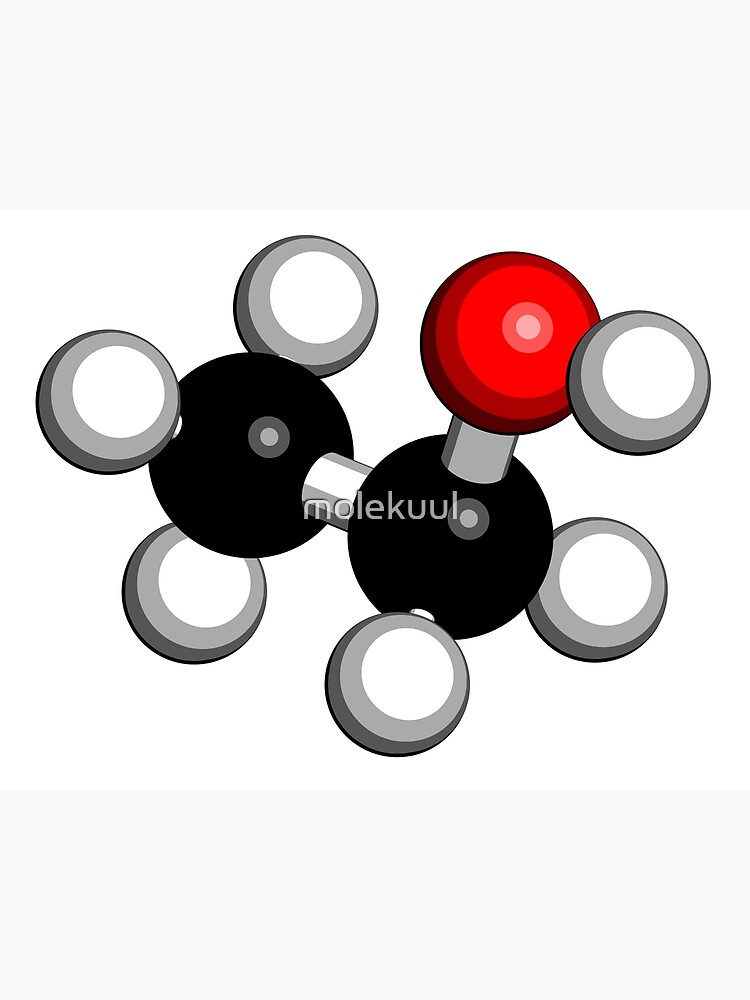This image displays a digital rendering of a molecular structure labeled as "Molekuul" (M-O-L-E-K-U-U-L) in gray letters across the center. The structure features two large black spheres central to the depiction, each containing a gray circle with a light gray interior. The left black sphere has three smaller white circles outlined in gray: one on the upper left, one on the upper right, and one on the bottom left, partially obscured as it goes behind the black sphere. A small gray tube-like connector on the right middle of this sphere links it to another black sphere positioned slightly lower to the right.

This right black sphere also contains a gray circle with a light gray interior and has three white circles with gray outlines connected to it: one at the bottom left, another just below the center on the right, which is partially obscured, and the third one on the upper side slightly to the right. Additionally, a small gray connector at the upper right of this second black sphere attaches to a red sphere featuring a smaller lighter red circle inside with a pink center. A white circle with a gray outline is also connected to the right of this red sphere. The detailed arrangement and specific connections between the spheres emphasize the complex and intricate representation of the "Molekuul" molecule.